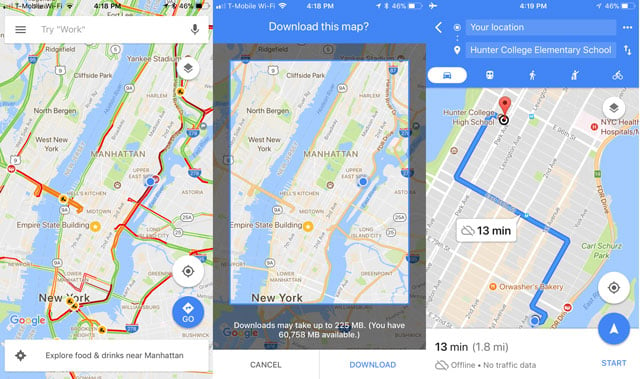Three side-by-side images from Google Maps showcase various functionalities for navigating the New York City area. The first image on the left displays a map of Manhattan, highlighting different routes with varying levels of traffic indicated by orange and red zones. Beneath this map, a box prompts users to "Explore food and drink near Manhattan." The center image features a download prompt with a blue border at the top labeled "Download this map." It details that the download will occupy up to 225 MB of space, with 60,758 MB available on the device. The rightmost image shows a pinned location in New York City and a blue route line indicating a travel distance of 1.8 miles, estimated to take 13 minutes.